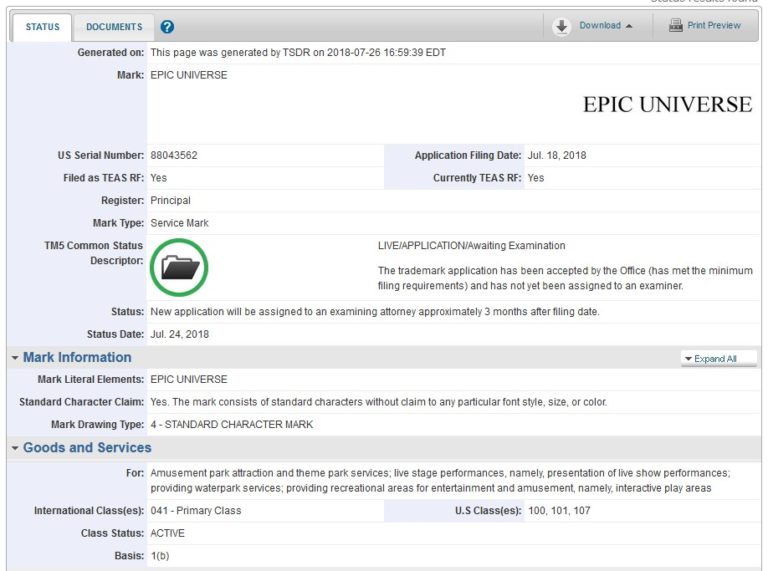In the upper left corner, a blue text reads "Status," adjacent to the word "Documents." At the top of the page is a long gray rectangle containing options such as "Download" and "First Preview." Below this, in black text, it states, "This page was generated by TSDR on 2018-07-26." Further down, the phrase "Mark: Epic Universe" appears, with "Epic Universe" in bold letters towards the right. 

To the right, a blue square highlights the "Application Filing Date" as "July 18th, 2018." Below, an image of a file within a green circle is displayed beside the text "TM5 Common Status." This section indicates that the "Status" is "New application will be assigned to an examining attorney approximately three months after filing date," with the status date noted as "July 24th, 2018."

In blue text is another category titled "Mark Information" followed by the mark literal elements, "Epic Universe." The section "Goods and Services" describes the services as "For amusement park attractions and theme park services, live stage performances, namely presentation of live show performances, providing water park services, providing recreational areas for entertainment, and amusement names interactive play areas." Finally, the classification "US Classes: 100, 101, 107" is noted within a blue square.